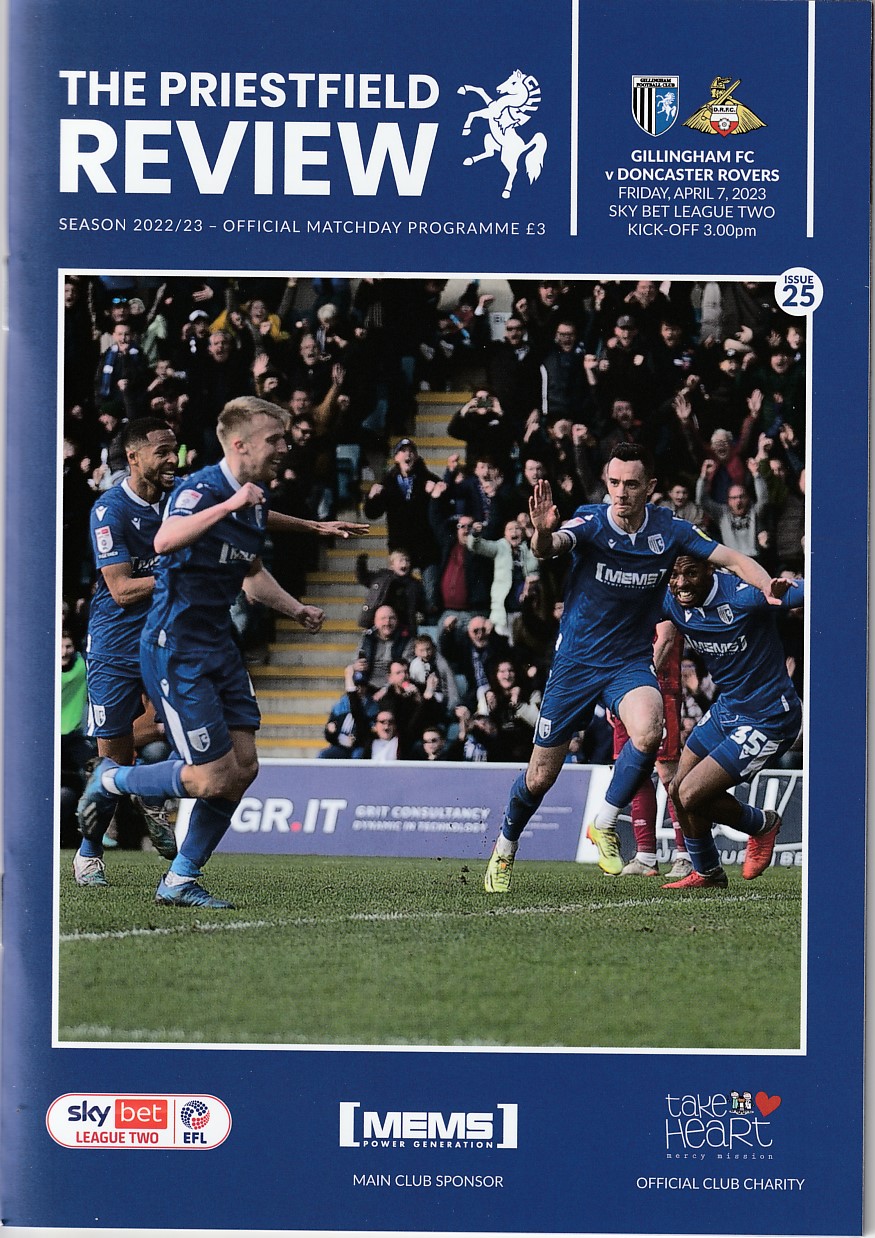The cover of the football program features a navy blue background with prominent white lettering. Central to the cover is a photograph capturing three football players from the same team, all dressed in blue kits with matching blue shorts and socks. Their boots distinguish them: one player sports blue boots, another yellow, and the third orange. The action shot shows the players running on the pitch with an enthusiastic audience behind them. At the top of the cover, the title "The Priestfield Review" is displayed alongside a horse emblem. Adjacent to the title are the crests of Gillingham FC and Doncaster Rovers, with match details: "Season 2022-23 Official Match Day Program, three pounds," "April 7, 2023, Sky Bet League 2, kickoff 3 p.m." Beneath the photograph, the program's sponsors are listed.